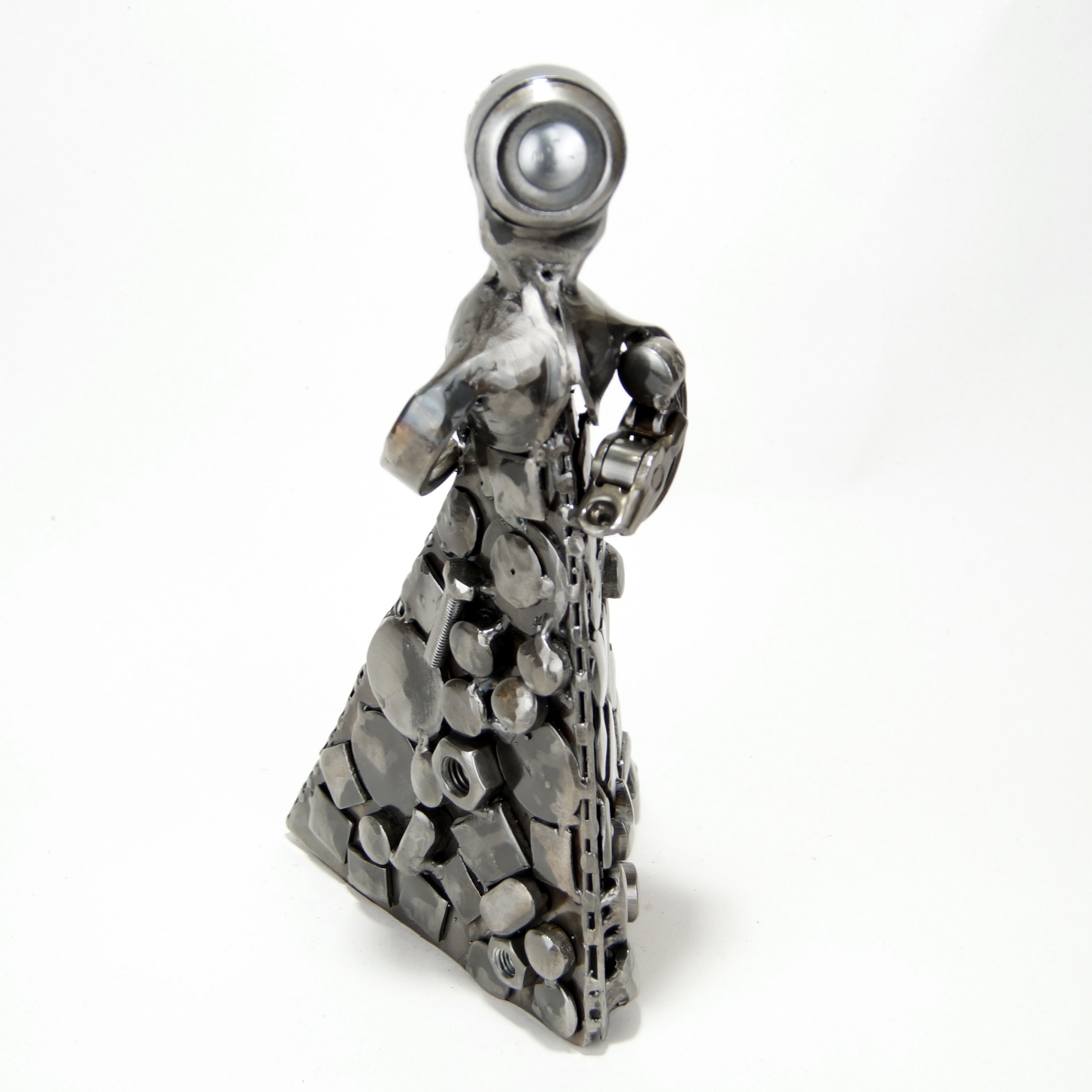This image showcases a detailed and artistic sculpture, constructed entirely from various silver metal components, such as screws, bolts, nuts, rods, and gaskets—elements you might commonly find in a tool kit. The craftsmanship transforms these mundane objects into a delicate figurine, resembling a woman adorned in a long, triangular-shaped dress, meticulously assembled from welded metal pieces. The figure's torso is fashioned from a larger chest-like piece with one arm extending forward as if offering a cup, while the other bends behind. The head of this figurine is represented by a circular element, resembling a nail or button, giving it a distinctive round shape. Overall, the sculpture is shiny and gray, with some darker hues, intricately combining round and squarish metal parts seamlessly melded together. The entire artwork sits against a stark white background, highlighting its intricate metalwork and the complex texture of its welded assembly.